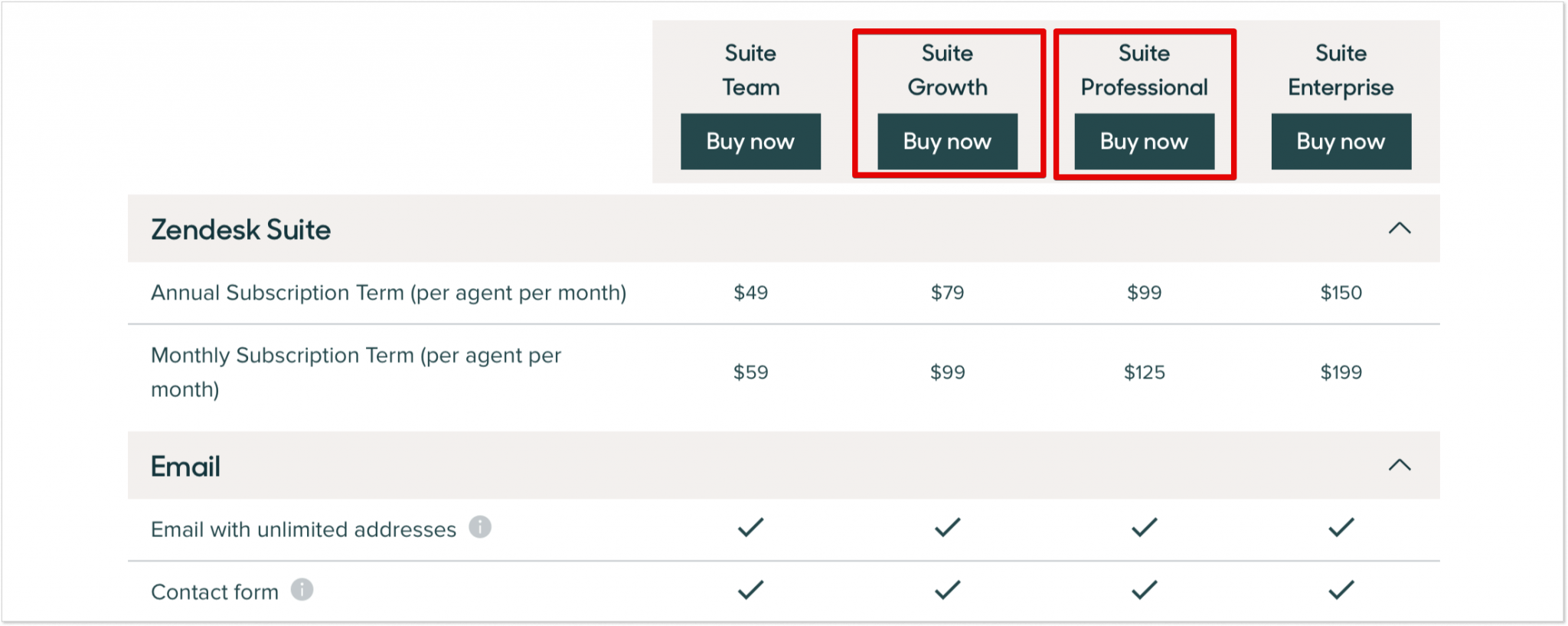This image is a screenshot of a subscription pricing page, with a predominant white background and no visible navigation bar for identification. The layout is structured into four columns at the top, all with grey backgrounds, each displaying different subscription options.

1. **Suite Team**: This column features a dark button labeled "Buy Now" in white text.
2. **Suite Growth**: A red square highlights this column, also with a "Buy Now" button.
3. **Suite Professional**: Another red square marks this column, which includes a "Buy Now" button.
4. **Suite Enterprise**: Featuring a "Buy Now" button as well.

Below these columns, there are two main headings, each with two rows of information:

- **Zendesk Suite**: This section has a pale grey background line and an up arrow on the far right. It includes:
  - Annual Subscription Term per Agent per Month: Prices listed under each column correspond to $49, $79, $99, and $150, respectively.
  - Monthly Subscription Term per Agent per Month: Prices listed under each column are $59, $99, $125, and $199, respectively.

- **Email**: This section also features a pale grey line and an up arrow on the far right. It includes:
  - Email with Unlimited Addresses: Each column features a tick mark indicating availability.
  - Contact Form: Each column features a tick mark indicating availability.

The screenshot efficiently compares the different subscription tiers, highlighting the Suite Growth and Suite Professional options for emphasis.